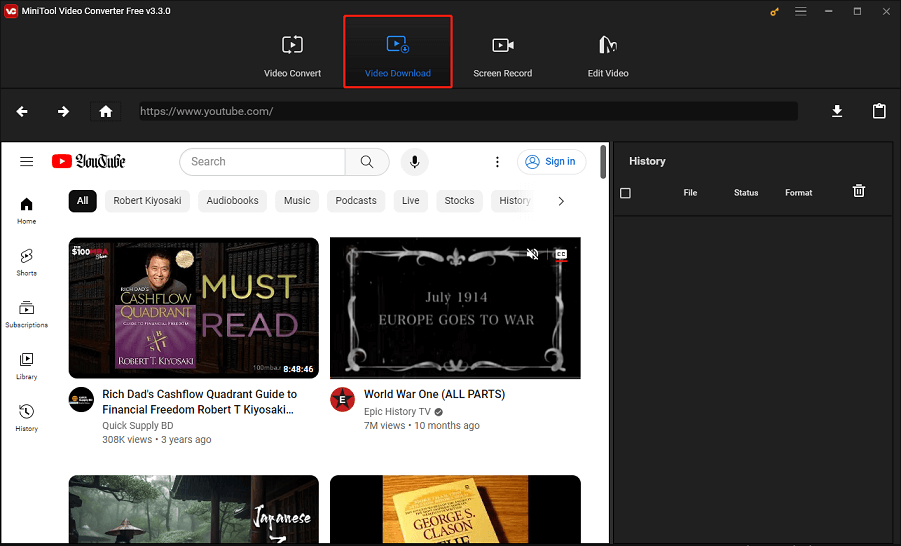The image is a screenshot of a computer screen displaying the "MiniTool Video Converter Free" software. The software's interface is set against a black background and features a distinctive "VC" logo at the top left corner. The upper portion of the interface has four primary options, arranged from left to right: "Video Convert," "Video Download," "Screen Record," and "Edit Video," written in small, blue, somewhat difficult-to-read text.

Beneath these menu options, the main body of the interface showcases a webpage called "Hard Read," designed in a sleek and stylish manner. This webpage appears to be a YouTube-like platform displaying four video thumbnails.

1. The first video thumbnail features a man standing next to a display titled "Rich Dad's Cash Flow Quadrant Guide: Financial Freedom by Robert T. Kiyosaki."
2. The second video is titled "July 1914: Europe Goes to War - World War I All Parts (Epic History TV)," which is hosted on the Epic History TV channel.
3. The details of the third and fourth videos are less clear but involve a Japanese theme in some capacity.